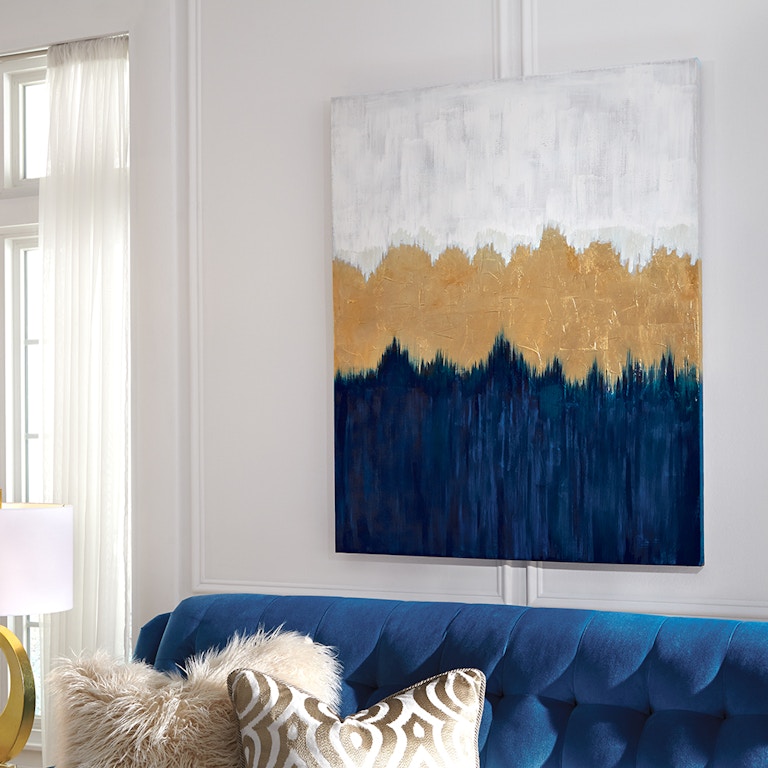This large square image showcases an elegantly styled living room with carefully placed furnishings and décor. Centered on the wall is a striking vertical canvas print, composed of three distinct sections: the top featuring vertical streaks of white and gray blending together, the middle adorned with a band of uneven gold that stretches horizontally, and the bottom showcasing navy blue streaked with light blue. This painting is hung between two sections of white wall panels that exhibit vertical ridges, adding texture to the background.

Below the painting, a luxurious brown, felt-covered sofa is visible, with the back cushion and two large square throw pillows prominently displayed. One pillow, positioned on the left, is a fluffy beige, while the other, on the right, exhibits an intricate gold and white pattern. To the left of the couch, a stylish gold lamp with a curved base and a simple wide white cylindrical lampshade stands beside the window. The window, partially obscured by semi-opaque white floor-to-ceiling curtains, hints at the sunlight streaming into the room, completing this thoughtfully arranged space, which may be part of an interior decorator's portfolio.